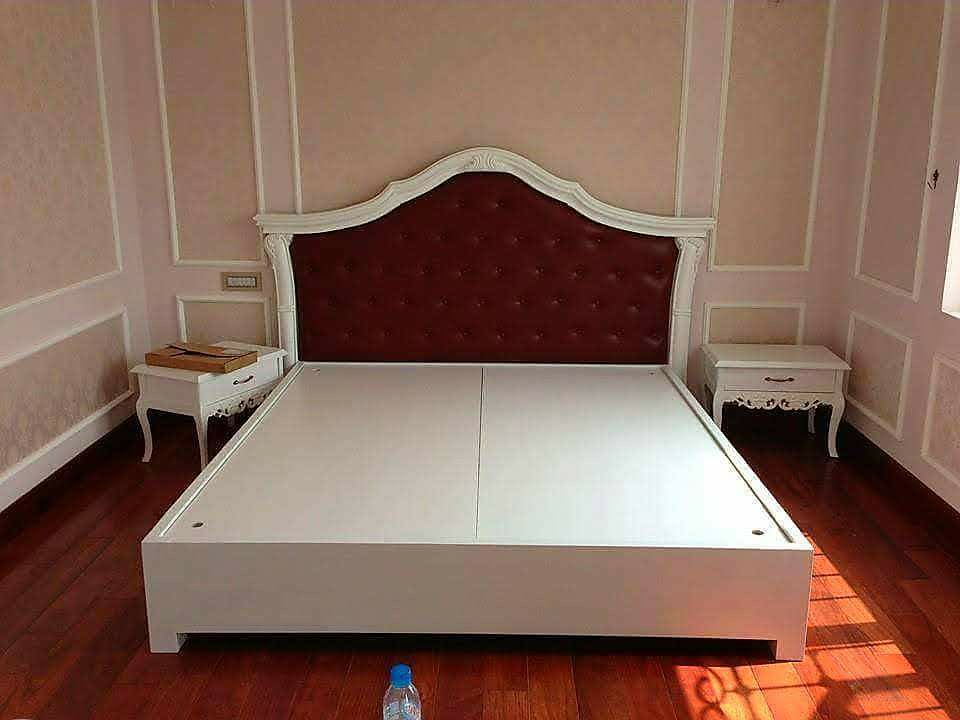This is a detailed photograph of a small bedroom with off-white walls featuring lighter-colored white panels and sections of pink wallpaper adorned with varying sizes of pink rectangles. The floor is a darker colored wood, resembling Brazilian cherry with a stained, non-glossy finish. At the center of the room is a large, rectangular white bed frame without a mattress, designed to cover the box springs with two separate pieces of wood that have small drill holes on the sides for easy lifting. The headboard of the bed is bordered in white with a dark brown, almost reddish, chocolate leather center, and is embroidered in white. On either side of the bed, there are elegant white nightstands. The nightstand on the left is slightly turned at a 45-degree angle and has a thin box with part of the cardboard lifted. The white nightstand on the right is plain. Additionally, there’s a plastic water bottle with a blue lid placed on the darker wood floor in front of the bed frame.